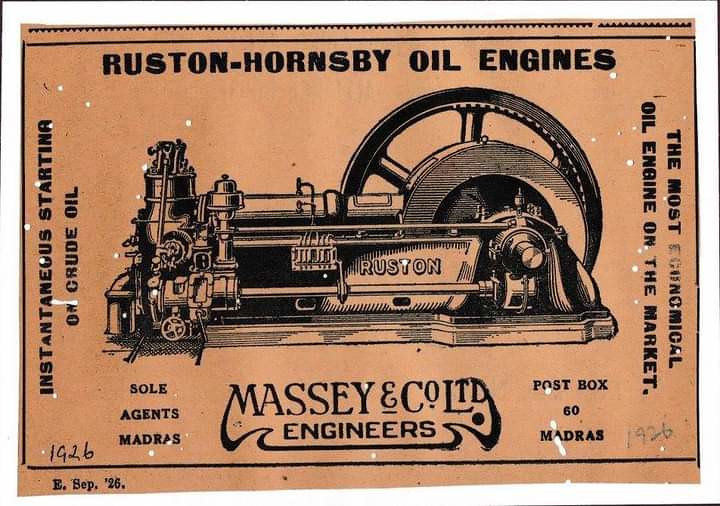The image is of an old-fashioned flyer with a predominantly orange background and a black line running along the borders. At the center, it prominently features an illustration of a vintage steam engine, which has a round wheel resembling a carriage wheel or tire rim. The top of the flyer displays the text "Ruston Hornsby oil engines" in bold black letters, followed by an inscription that reads "the most economical oil engine on the market." The phrase "Instantaneous starting on crude oil" is also visible on the left side of the engine illustration. Below the engine, the text reads "Massey E. Co. Ltd. Engineers" and "Sole Agents Madras," alongside "Postbox 60, Madras." The bottom left corner of the flyer has the handwritten number "1926," and printed beneath that is "E. CEP 25." The flyer is perforated with white dots scattered across it, suggesting age or wear.